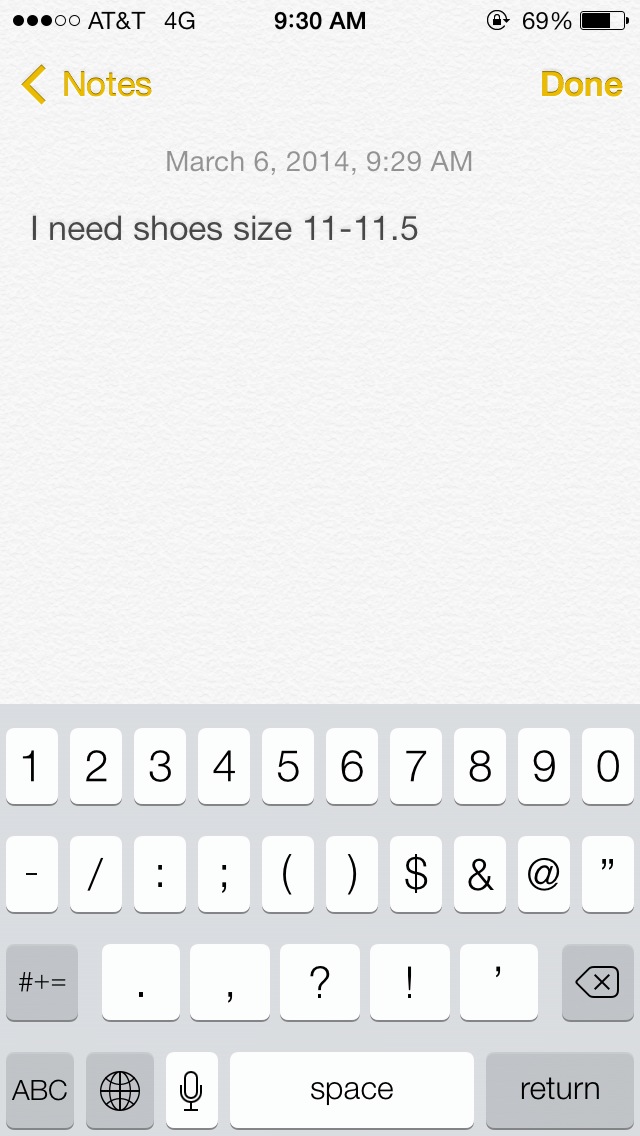The image depicts a screenshot of the Notes app on an iPhone. At the top of the screen, the status bar shows "AT&T 4G" on the left, the time "9:30 AM" in the center, and a battery level of "69%" on the right. The main part of the screen features a note titled "Notes done" created on March 6, 2014, at 9:29 AM. The content of the note reads: "I need shoes size 11 to 11.5." The background of the note has a faux paper texture with the text in black. Below the note, the iPhone's digital keyboard is visible, featuring numerical and special characters in white and gray, with a few black highlights. The keyboard includes standard keys like numbers, various punctuation marks, and symbols, along with special function keys such as "ABC," a globe icon for language settings, a microphone, space bar, and return key. The overall appearance conveys a typical use of the Notes app to jot down a reminder about shoe sizes.